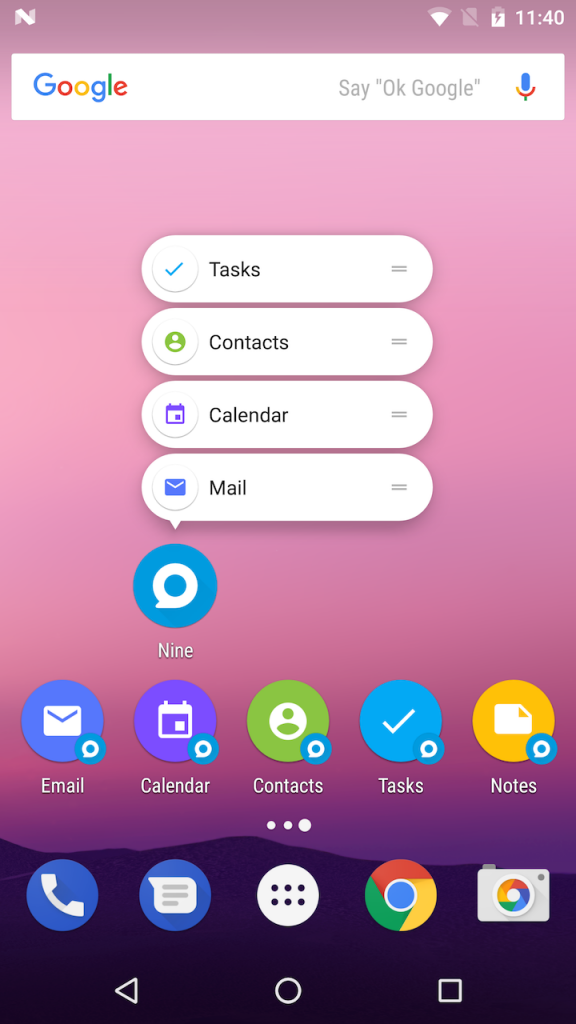The image depicts the front screen of an Android phone, showcasing a variety of elements in a detailed and organized layout.

At the very top, there is a status bar displaying the current time, 11:40, alongside various icons. These icons indicate the phone is charging, with approximately three-quarters of its battery remaining, and show a strong network connection. To the left, an "N" logo is visible, likely representing a notification or NFC connection.

Below the status bar is a Google search bar. It features the Google logo on the left and a microphone icon on the right, with the prompt "Say, 'OK Google'."

The background image of the screen resembles a picturesque scene at dawn or dusk, with a blend of pink and purple hues over a horizon lined with dark, silhouetted mountains.

Centered prominently on the screen are four essential options: "Tasks," "Contacts," "Calendar," and "Mail," each accompanied by its respective icon. Directly beneath these options, a grid of nine app icons is neatly arranged. The applications include email, calendar, contacts, tasks, and notes, all adorned in various colors such as blue, purple, and yellow.

Towards the bottom of the screen are five primary icons in a fixed dock, from left to right:
1. A blue telephone icon with a white handset, representing the phone app.
2. A messaging icon.
3. A settings icon, depicted as a white circle with six dots.
4. The Google Chrome icon.
5. A camera icon.

Finally, at the very bottom of the screen are the traditional Android navigation buttons: a triangle for "Back," a circle for "Home," and a square for "Recent Apps."